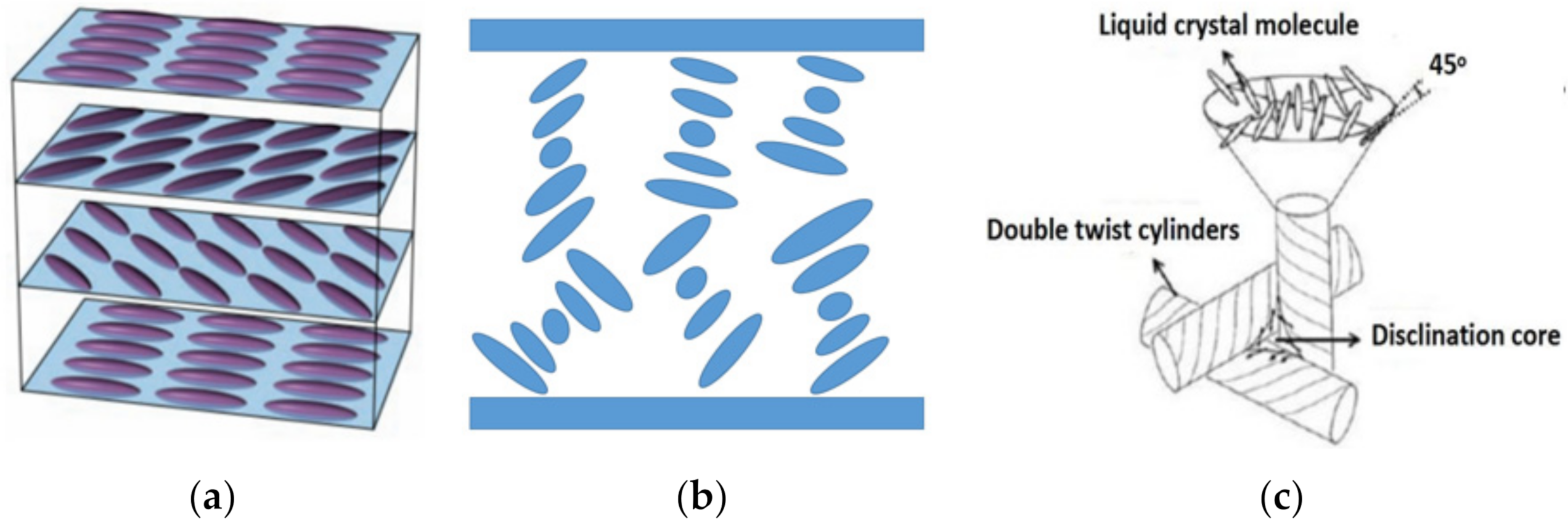This scientific diagram consists of three parts, labeled A, B, and C. In Image A, we observe an artist's depiction of a four-tiered metal shelf. Each tray on the shelf features a blue plate with purple dots. The dots on the first and fourth trays are arranged horizontally, while the second and third trays have them in diagonal patterns. Moving to Image B, the diagram presents a white backdrop adorned with light blue ovals and a blue border that runs along the top and bottom edges. The ovals are arranged at various angles, creating a dynamic visual effect. Finally, Image C displays a black-and-white illustration of a liquid crystal molecule. This image shows a funnel with a striped base, and labels indicating "double twist cylinders" and a "disclination core." Arrows point to specific areas of the base and the middle of the cylinder, highlighting key components. Together, these images illustrate aspects of polymers, multi-phase liquid crystal filters, and single-layer polymer templates.